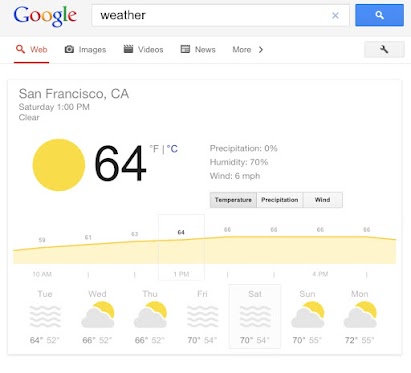This image is a detailed snapshot taken from Google, displaying the current weather for San Francisco, California. The time shown is Saturday, 1 p.m., with a current temperature of 64 degrees Fahrenheit. The interface features a comprehensive weather forecast for the upcoming week, spanning from Tuesday to Monday. 

Centrally, a line graph outlines the temperature fluctuations expected throughout the day, covering the period from 10 a.m. to 5 p.m. Accompanying data points include wind speed at 6 miles per hour, humidity at 70%, and a precipitation probability of 0%, indicating no rain.

At the top of the image, the familiar Google logo is positioned in the top left corner adjacent to a search bar, which indicates the search term "weather." To the right of the search bar is a blue search button adorned with a magnifying glass icon. This detailed Google search interface provides a clear and concise summary of the current and upcoming weather conditions for San Francisco.